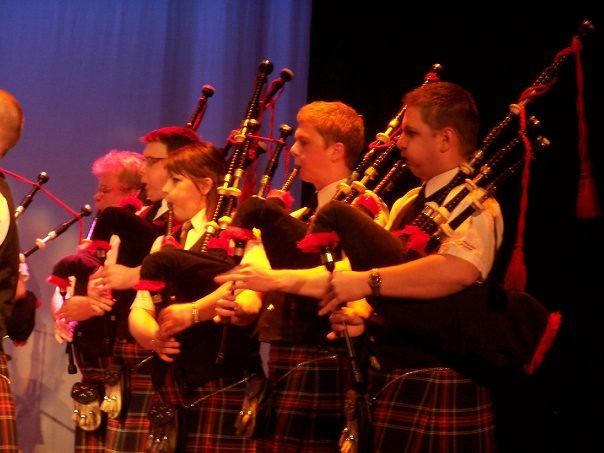The photograph captures a theatrical performance of bagpipe players on a well-lit stage. The scene is set against a backdrop that transitions from a bluish-purple stage curtain on the top left to a dark brown background on the right. Five musicians are prominently positioned in a diagonal line from the center right to the back left. All five are clad in traditional plaid kilts, white short-sleeve shirts, and black vests, with sporrans hanging in front. Their bagpipes are distinguished by dark brown pipes adorned with red and gold fixtures. Notably, red tassels are tied to the pipes, enhancing their visual appeal.

Among the players, there are three men and two women: on the far right, a male with a watch on his wrist; next to him, a redheaded man; in the center, a brunette woman with a watch; followed by a man wearing glasses; and on the far left, a woman with glasses. Additionally, glimpses of another group of bagpipe players can be seen on the left edge of the image, indicating the presence of at least two more musicians, similarly dressed and positioned slightly out of the frame. The lighting accentuates the performers, capturing the vibrant atmosphere of the stage.